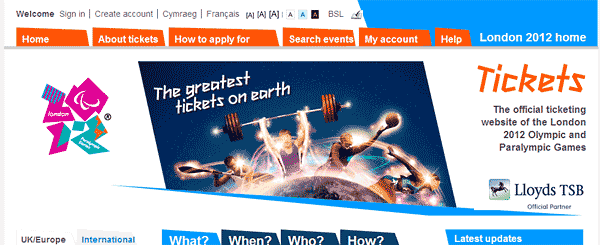This is a screenshot of a web page. At the top of the page, there is a navigation bar with several selectable options arranged from left to right. The options include "Welcome, Sign in," "Create Account," "CYMRAEG," "Française," three different sized 'A's for text size adjustment, and "BSL." To the right of these options, there is a blue banner. 

Below this navigation bar, another row features links with an orange background and white lettering. These links are labeled "Home," "About," "Tickets," "How to Apply For," "Search Events," "My Account," and "Help." In the same blue banner on the right, there is text that reads "London 2012 Home" in white.

Beneath this section on the left-hand side, there are various shapes in pink, green, and blue colors with a registered trademark, though the exact nature of these shapes is unknown. Adjacent to this, there is an image with the text "The Greatest Ticket on Earth." This image depicts an athlete lifting weights, another throwing a basketball, and representations of other sports, all positioned atop a globe with light trails resembling light painting.

On the right-hand side, the word "Tickets" is prominently displayed in orange. Underneath this, in smaller black print, is the description: "The official ticketing website of the London 2012 Olympic and Paralympic Games." Beside this, the text "Lloyd's TSB" is visible. Towards the bottom, links labeled "UK," "Europe," and "International" are available, accompanied by options for "What," "When," "Who," and "How." On the far right-hand side, there is a section titled "Latest Updates."